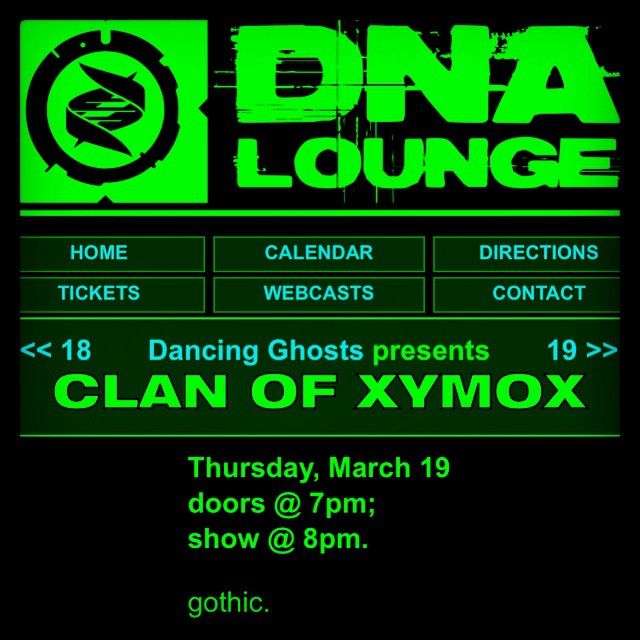The image depicts a screenshot of a website advertising an upcoming event at DNA Lounge. The background is solid black, providing a stark contrast to the various elements in the image. At the top left corner, there is a green square logo followed by the text "DNA Lounge" in green. Below this, there is a sequence of menu items presented in light green rectangles: "home," "calendar," "directions," "tickets," "webcast," and "contact," all centrally aligned.

Prominently displayed in the middle of the image, text announces "Dancing Ghosts presents Clan of Zymox" with event details beneath: "Thursday, March 19, doors at 7 p.m., show at 8 p.m." An arrow pointing to the left, labeled "18" in lighter blue, is also visible on the left side. Additionally, the term "gothic" appears twice, once as "dot gothic" and once as just "gothic," both in green text. This detailed graphical layout clearly aims to inform visitors about the scheduled show at DNA Lounge.